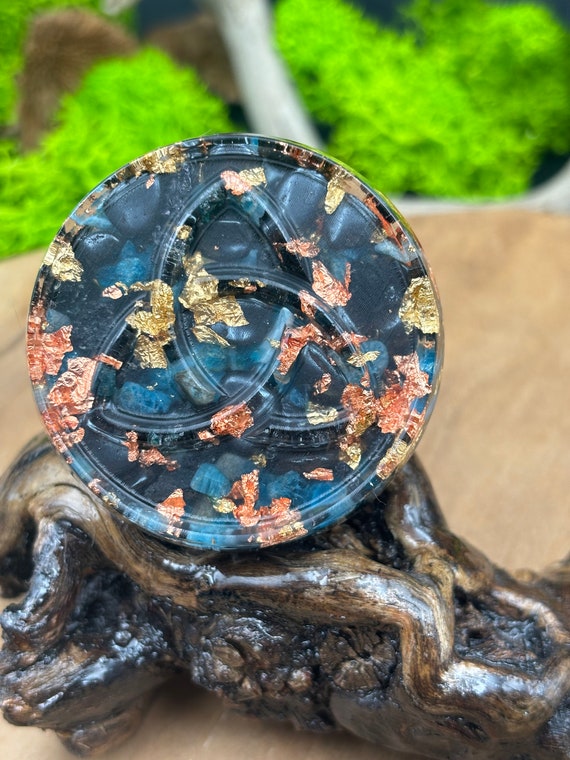The image captures a detailed close-up of a sophisticated artifact—a black plate that appears to be crafted from a composite material and is embellished with flakes of gold and copper leaf. The plate is round with a defined rim and features three interlocking, oval-shaped symbols geometrically aligned at its center, reminiscent of one of Led Zeppelin's iconic symbols. The surface of the plate showcases splotches of gold and copper leaf, giving it a luxurious and intricate appearance. This ornate plate is elegantly displayed on a stand made from a polished and stained piece of driftwood, with its gnarled and knotted texture reminiscent of a bonsai tree trunk. The background of the image is slightly out of focus, showcasing bright green foliage, what seems to be a white tree branch, and some brown, clay-like elements, possibly suggesting that the plate is part of a bonsai tree planting. The rich colors and textures of the plate and its stand create a visually striking centerpiece against the natural background.